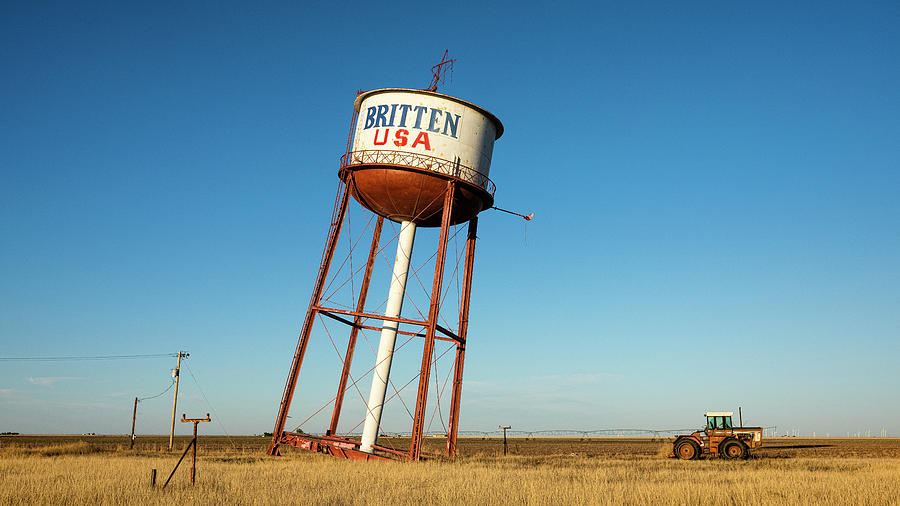In this image, set against the clear, bright blue sky of a sunny day, we see a dramatic, leaning water tower that appears to be mimicking the iconic Leaning Tower of Pisa. The tower, which stands amidst vast farmland with tall yellow grass, has a round container at the top, marked with the words "Britain USA"—'Britain' is written in blue, and 'USA' in red. This peculiar structure is supported by a white pole and four legs at the corners. The horizon is flat and almost empty, save for a few utility poles and a tractor positioned precariously underneath the leaning tower. Despite its pronounced tilt to the right, no one nearby seems concerned about the tower's stability.